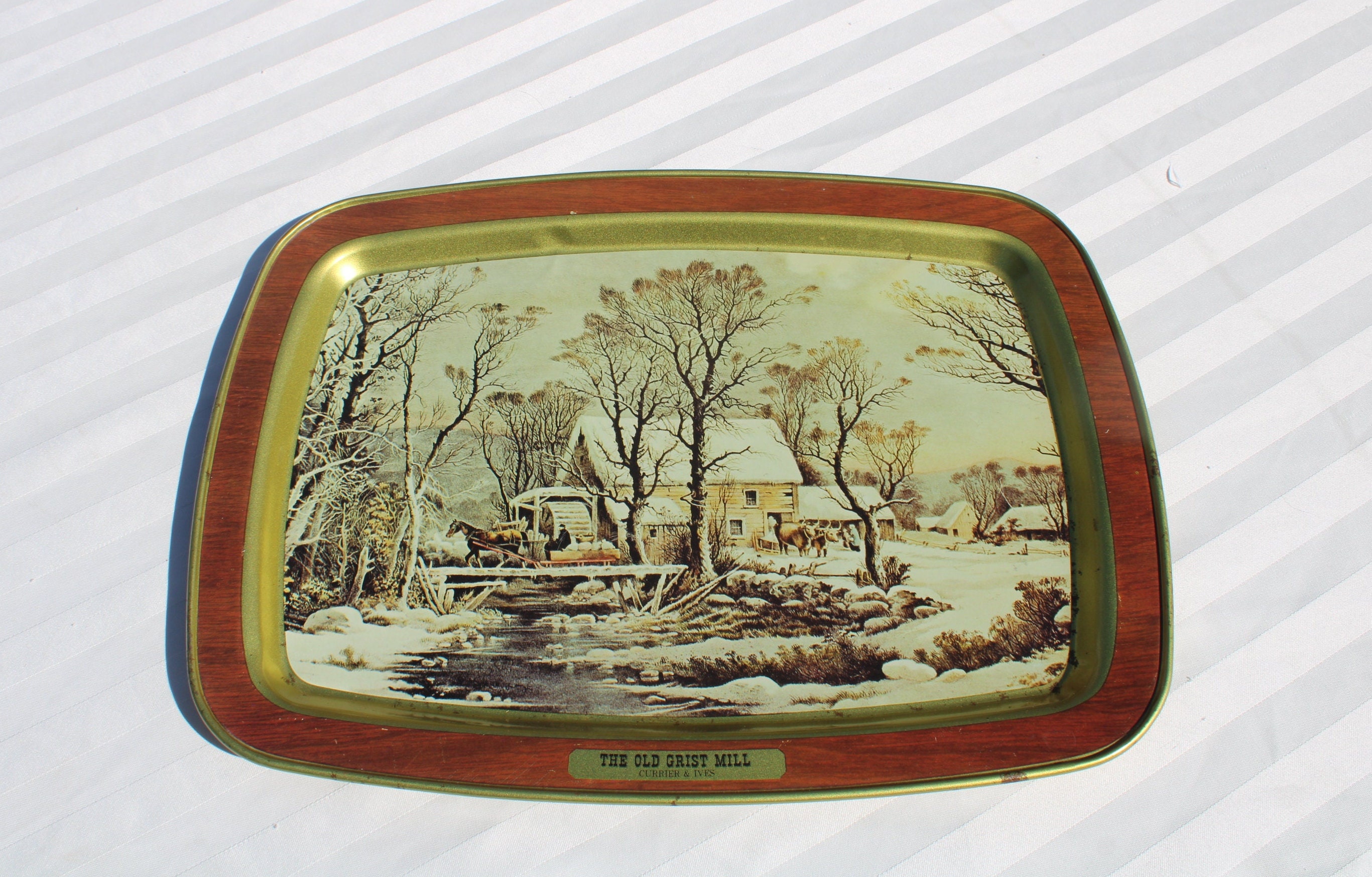This image depicts a vintage decorative tray featuring a picturesque winter scene centered around an old wooden mill labeled "The Old Grist Mill" on a gold plate. The snowy landscape showcases snow-covered roofs, trees, and ground, with a frosty creek running through the scene. The mill is accompanied by horses and a serene figure sitting nearby, conveying a tranquil and peaceful atmosphere. The artwork is bordered by a raised gold edge, which is further enclosed by a band of wood that also holds the gold text label. The tray sits on a table adorned with gray and white items.